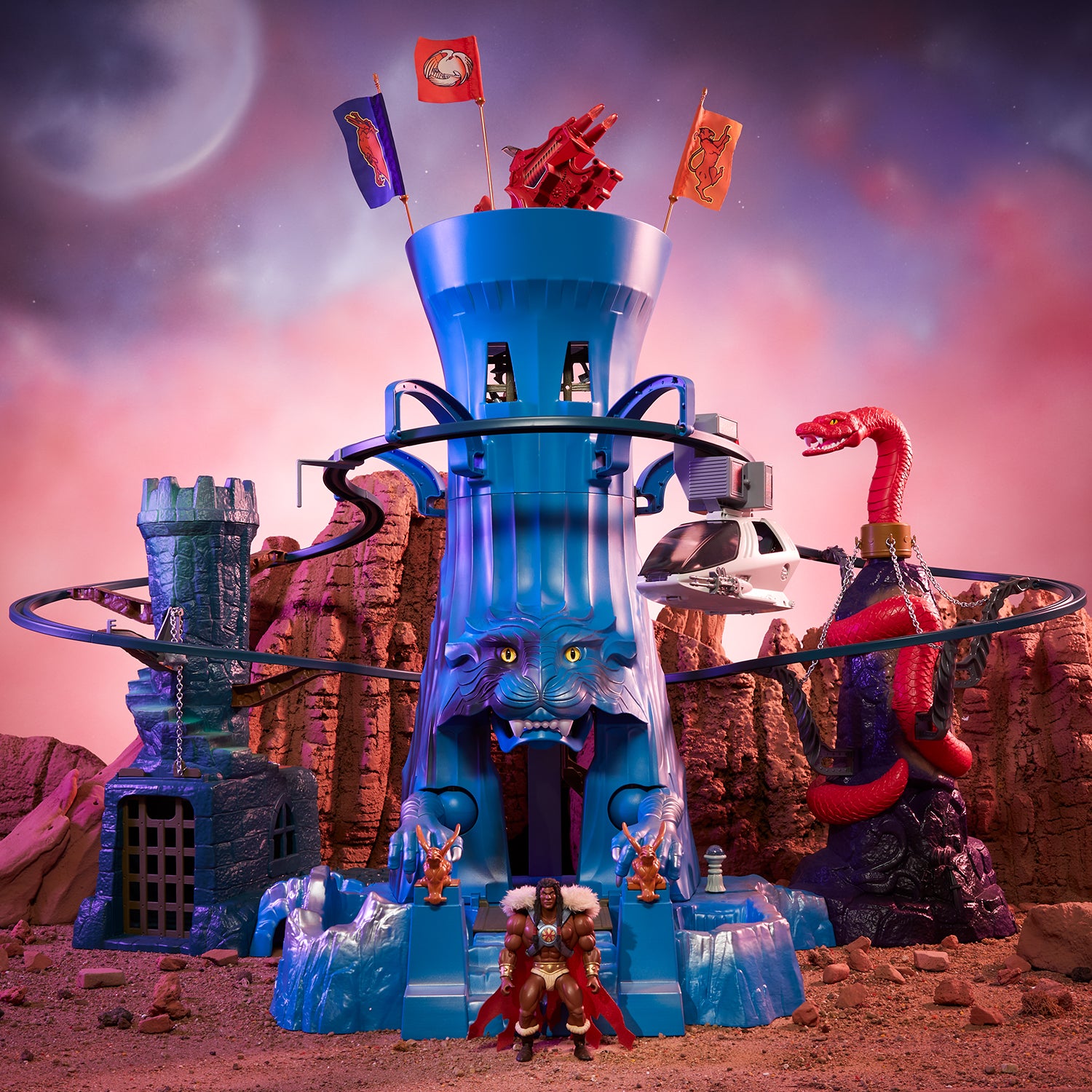This rectangular image, slightly taller than it is wide, showcases a dramatic playset scene designed to resemble an action-packed desert landscape. The rocky, reddish-brown ground extends beneath an intricately detailed blue toy structure, resembling a tower adorned with flags and encircled by a railing that supports a sky cab. This towering blue statue boasts a wild feline face with yellow eyes and a gritted grin, ominously guarding the scene. Descending from its steps is an imposing action figure with bulging muscles, dressed in wrestling shorts with a fur coat, and sporting dark hair.

To the statue's right, a red snake coils around a brownish-purple formation, adding to the sense of peril. Another smaller blue tower stands to the side, contributing to the complex layout. In the sky above, shades of pink, white, purple, and blue blend elegantly, crowned by a solitary moon in the top left corner, completing the vivid, imaginative backdrop of an adventurous children's playset display.